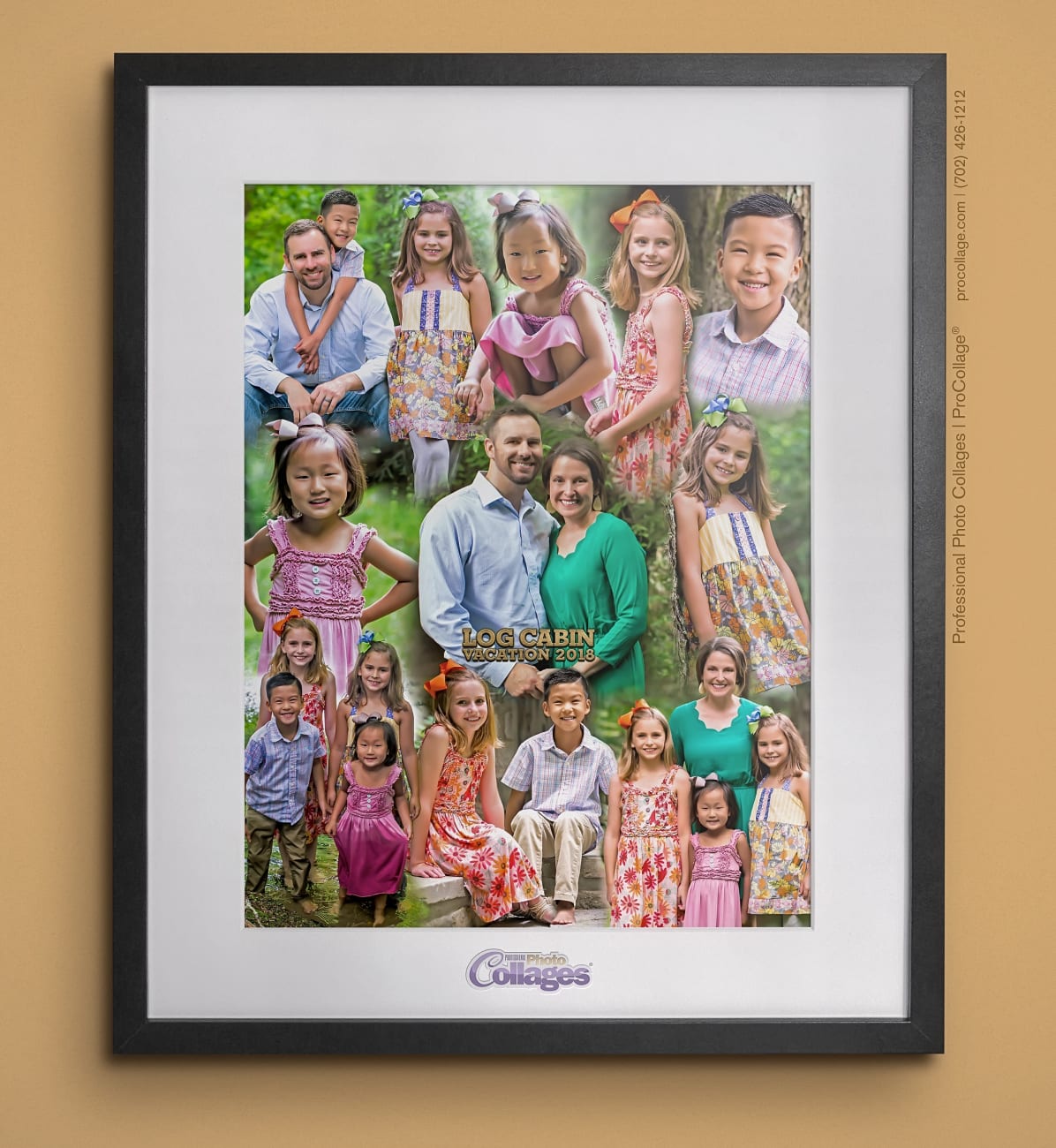This image depicts a professionally framed family photo collage from ProCollage.com, with the frame featuring a sleek black border and white matting. The collage comprises various family photos centered around a couple, who are flanked by four children of diverse ethnic backgrounds, including Asian and Caucasian. The collage captures individual and group shots of the children, suggesting the family may have adopted some of them. All photos appear to be taken during the spring or summer, evident from the children's sleeveless dresses and the lush greenery in every background. The collage is displayed against a gold-toned, beige wall, and includes text detailing, such as "Log Cabin Vacation 2018," highlighting a memorable family event.